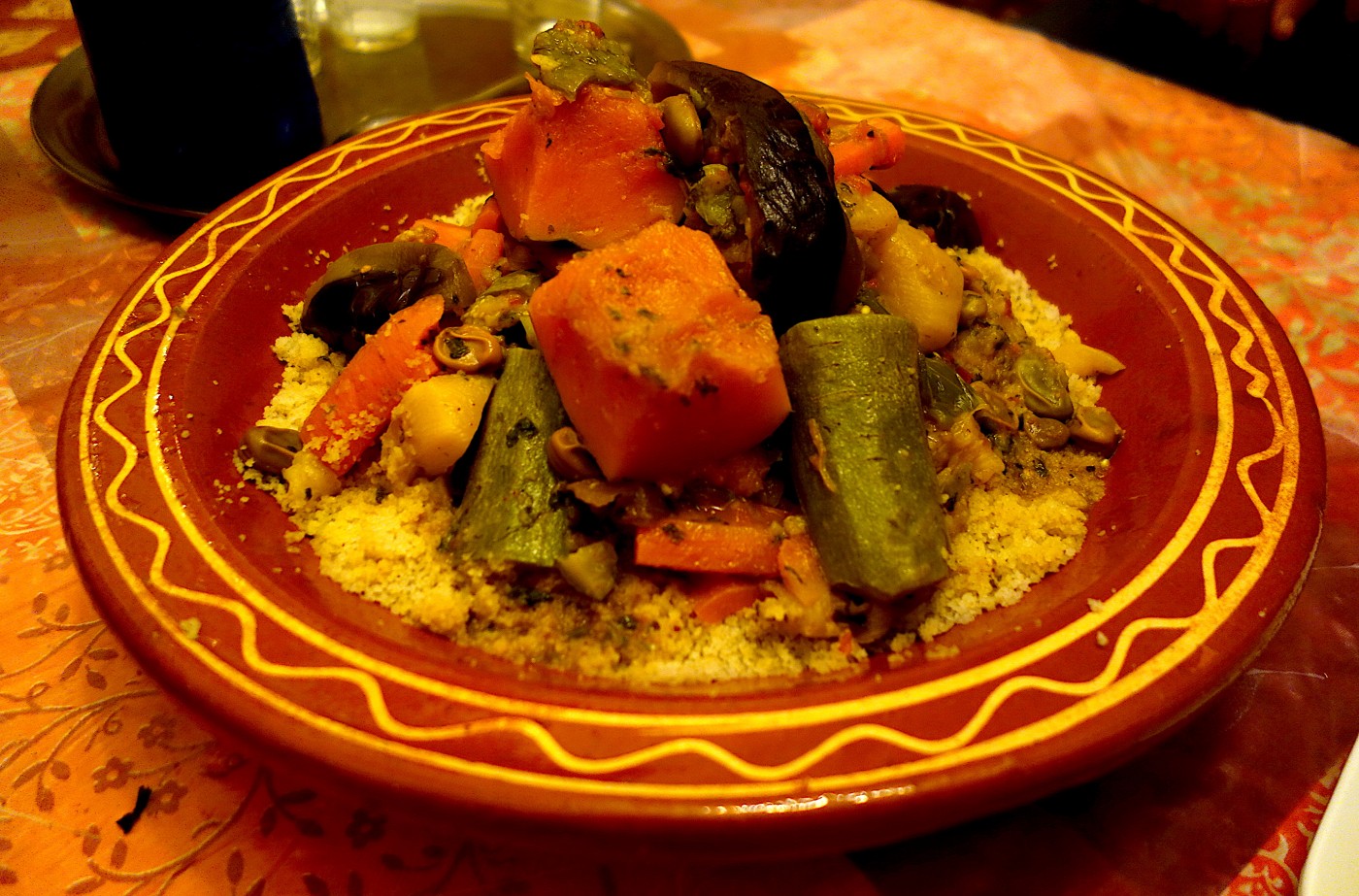A close-up photograph captures a vibrant bowl of food, likely taken indoors under warm, orange-hued lighting. The shallow, wide bowl appears to be made of pottery, featuring a red exterior adorned with either white or yellow geometric designs around its rim. The contents of the bowl seem to be couscous, topped with a medley of vegetables including light orange chunks that resemble yams, thick green pieces, and possible slices of eggplant. 

The bowl is placed on a tablecloth with a floral pattern, adding a touch of homeliness to the scene. In the background, a metal plate or tray is visible, holding several small bottles and a larger one, suggesting a setting that could be a cozy restaurant. Overall, the image portrays a warm and inviting dining atmosphere.